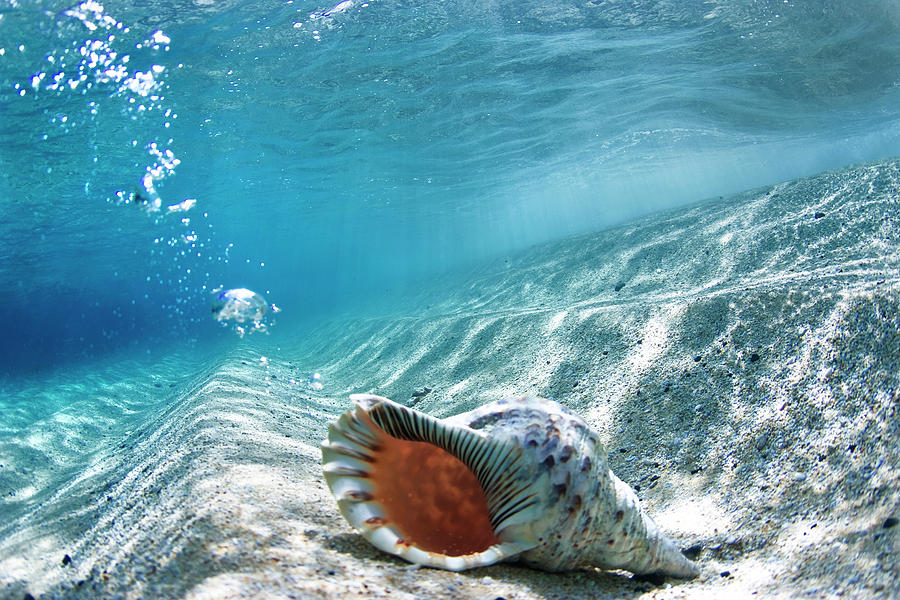The underwater photograph captures a serene and beautifully lit scene of a large conch shell resting on the sandy bottom of a shallow ocean. In the center bottom of the image, the shell with its multi-colored patterns of black, purple, and white is positioned with its opening facing toward the viewer, suggesting it might be inhabited by a crab, as small air bubbles rise from it. The white, gently cascading sand formations create a tiered, wave-like effect that slopes downward from the top right. Surrounding this tranquil setting, shafts of sunlight filter through the clear, bright blue water, illuminating the scene. The water darkens slightly in the left center of the image, adding depth to the otherwise brilliantly lit underwater beach.